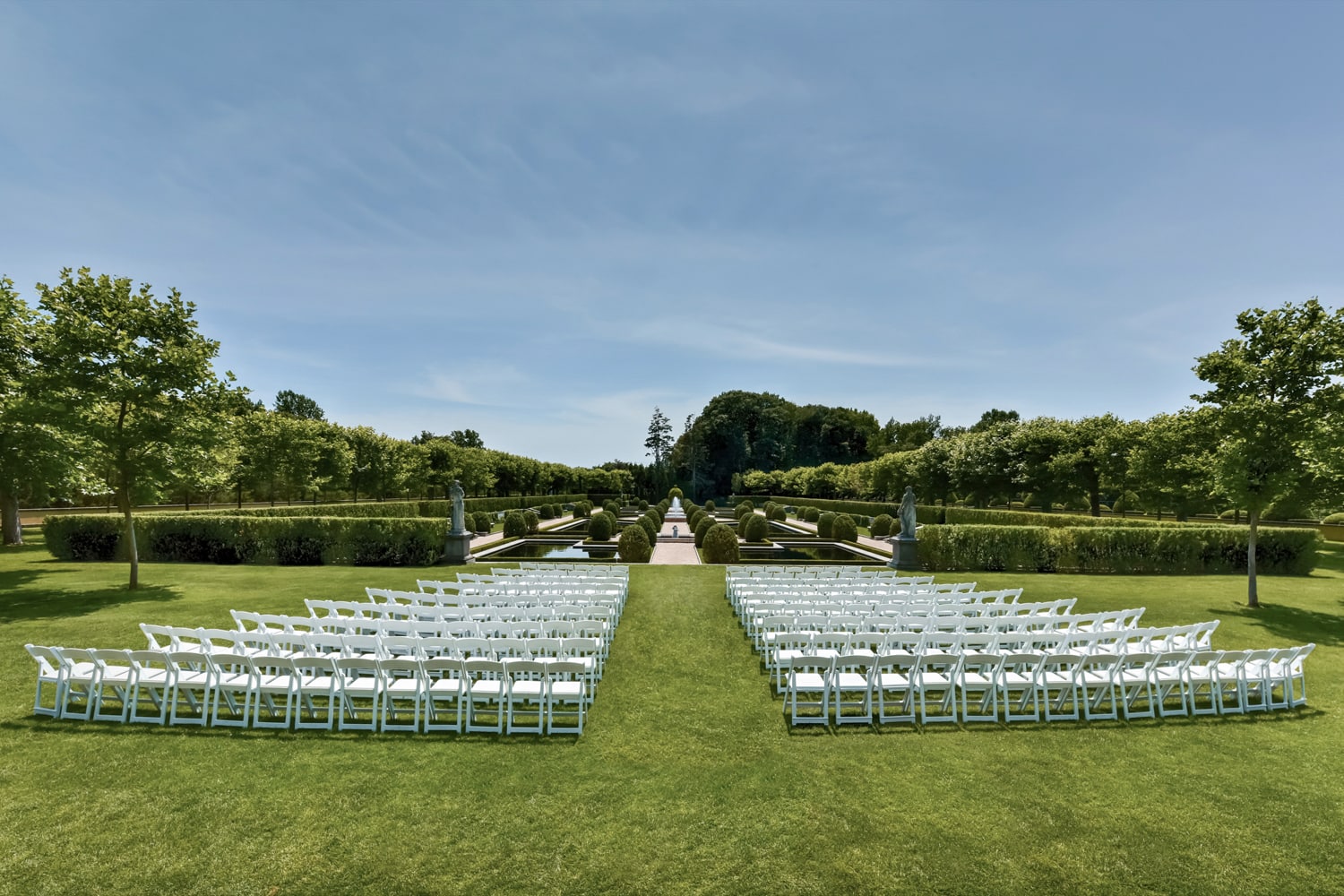The outdoor photograph depicts a large, well-maintained park or estate garden in late spring or summer, characterized by vibrant greenery and a clear blue sky with minimal clouds. At the forefront, approximately ten to twelve rows of evenly spaced, white foldable chairs are set up on a lush green lawn, forming two sections divided by a central aisle. This arrangement suggests preparation for a significant event, possibly a wedding. Flanking the chairs are two prominent trees, and, beyond the seating, a manicured hedge encloses a pathway that leads to water features with paved sections and round-shaped topiaries. The scene extends outward with more trees and possibly small statues at the ends of the hedge, adding to the picturesque and serene atmosphere of the setting.